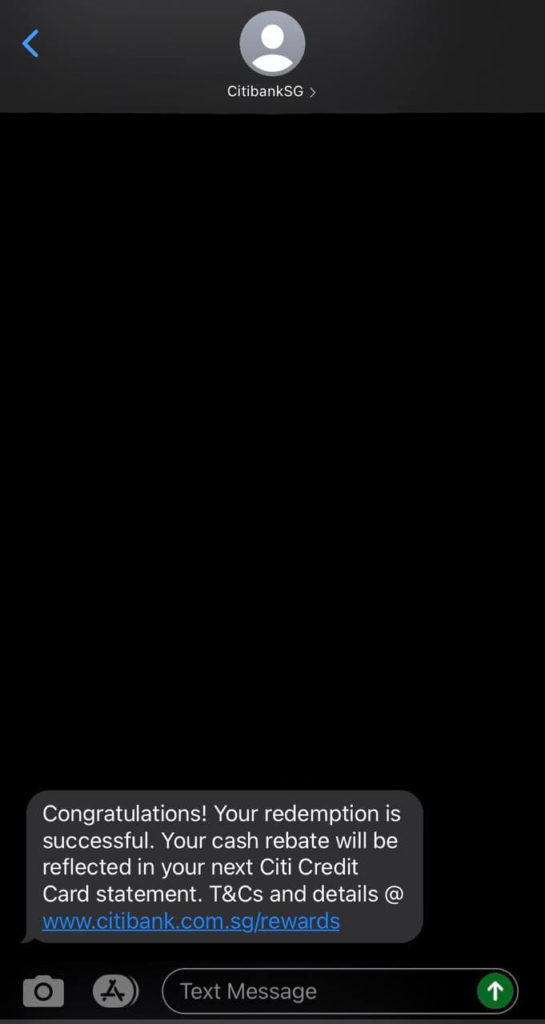The image features a dark background with a gradient from dark grey at the top. In the top-left corner, there is a blue arrow pointing to the left. Adjacent to this, on the right, is the text "CITIBANKSG", with a grey circle above it containing a white silhouette of a person, resembling a profile picture placeholder.

Toward the bottom of the image, a congratulatory message reads, "Congratulations! Your redemption is successful. Your cash rebate will be reflected in your next Citibank credit card statement. Terms and conditions and details at www.citibank.com.sg." The word "Rewards" is highlighted in blue within this section.

At the very bottom, there is a green circle with a white upward arrow inside it, accompanied by a small "A" to the left and a camera icon nearby.